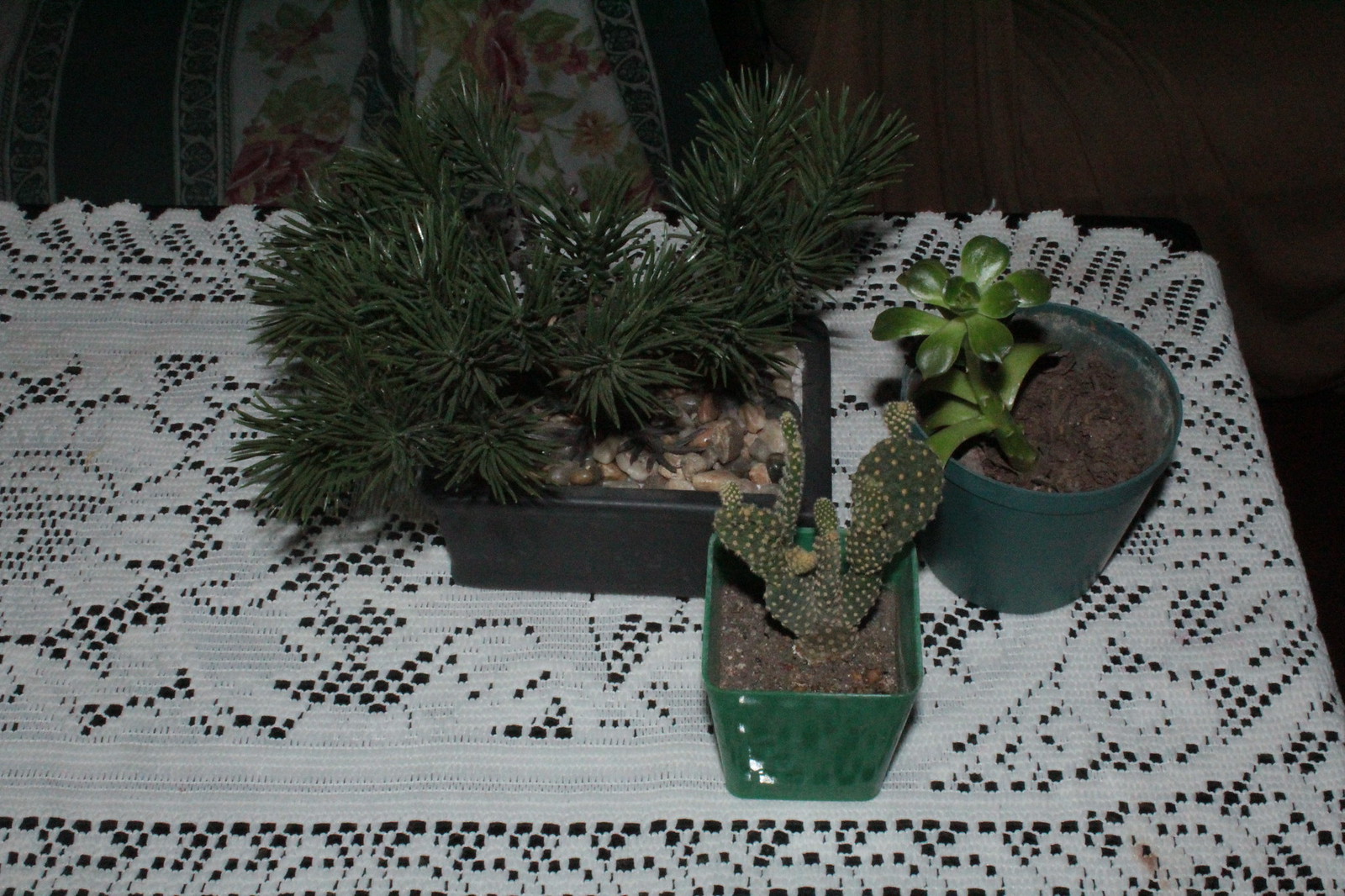This is a color, horizontal photograph depicting the interior of a dimly lit room, with the focus on a rectangular table covered by a white tablecloth. Centered on the table are three distinct potted plants. The planters vary in shape and color: one black rectangular pot containing rocks and soil, housing what appears to be a succulent with sharp, pointy leaves; a green ceramic container with a cactus; and a rounded green plastic container holding another cactus that is shaped like a green flower, characterized by its round, softer leaves. The room's dark ambiance is highlighted by a flash from the camera that captured the image. Visible in the background are a wooden floor, a floral blanket or rug with pink flowers, and the arm of a brown sofa. There might also be a chair and possibly a wood grain wall, inferred from the overall setting.